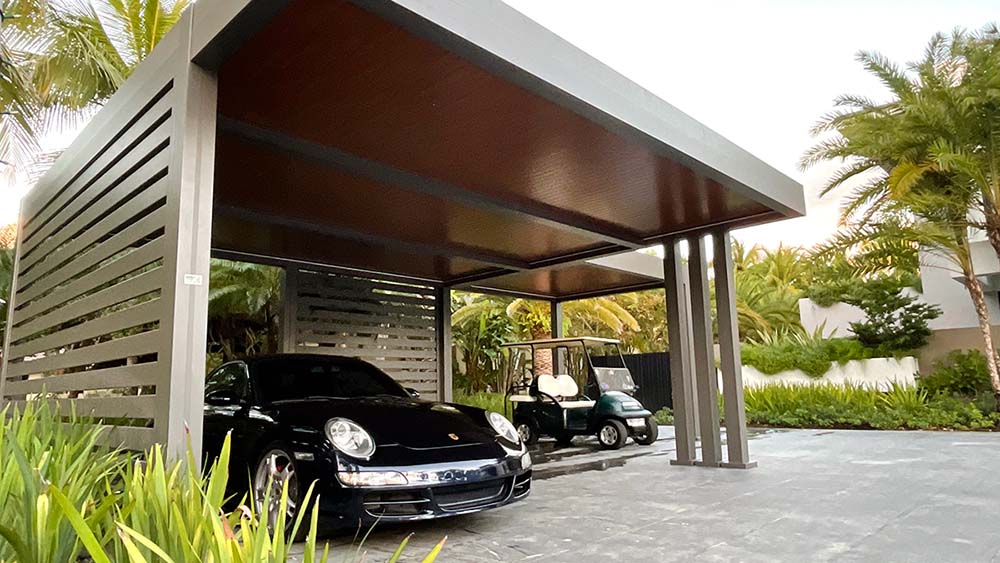The image is a rectangular outdoor scene, wider than it is tall, set in what appears to be a tropical region. It features an elegant silvery copper structure, reminiscent of a fancy carport with slotted walls and a flat ceiling. Beneath this polished canopy, a sleek black sports car with large round headlights is parked. Adjacent to it, under a smaller segment of the carport, a black golf cart with a white roof rests. To the left of the carport, lush greenery grows at the bottom, adding vibrant foliage to the scene. Palm trees with their long leaves appear prominently, both shooting up from the right-hand side towards the top corner and stretching out from the top left. The background shows a modern, blocky building with a cream and brown façade. The scene also includes notable tropical vegetation, including long grasses and bushes. The setting suggests a high-end location, highlighted by the pristine cement floor of the carport and the overall refined aesthetic of the environment, under a light-colored sky.